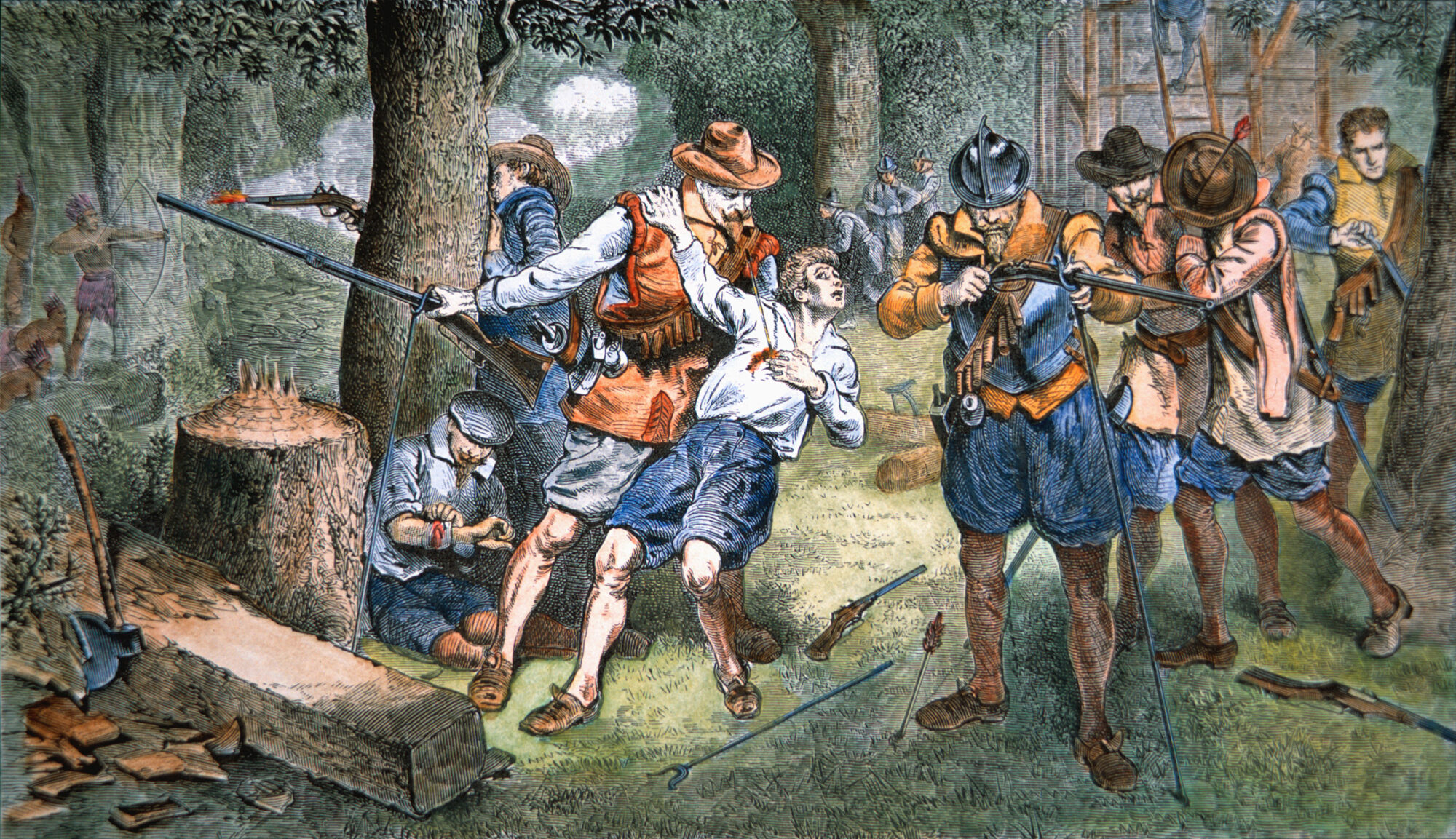The image depicts an old painting or detailed computer-generated rendition of a historic battle scene set in a dense forest, possibly during the era of early American exploration or the Civil War. The foreground is dominated by a group of men, predominantly dressed in white long-sleeve shirts, orange tunics, and blue or beige puffed shorts, some of whom wear silver or brown hats reminiscent of cowboy hats. Their feet are clad in simple brown loafers, and several are holding or loading rifles and muskets, pointing towards an unseen enemy.

A dramatic moment is captured at the center, where a young boy in a white shirt, with two arrows protruding from his chest, collapses backward into the arms of a man in an orange tunic, who is trying to support him. Blood is visible on the boy’s chest, indicating he has been critically wounded. Around them, other men are attending to their own injuries or continuing their struggle, amidst a chaotic scattering of arrows and falling wooden debris. On the left side of the image, a piece of wood with an embedded axe and a nearby tree stump suggest ongoing efforts to chop down trees, possibly for building a fort or settlement, as indicated by a partially constructed structure visible in the background.

In contrast, the background features Native Americans with bows and arrows, hiding among the trees, actively engaging the explorers in combat. The tension of the battle is palpable, with arrows lodged in the ground and several Native Americans aiming their arrows toward the men. The painting captures a moment of intense conflict and cultural clash, blending historical details with dramatic visual storytelling.